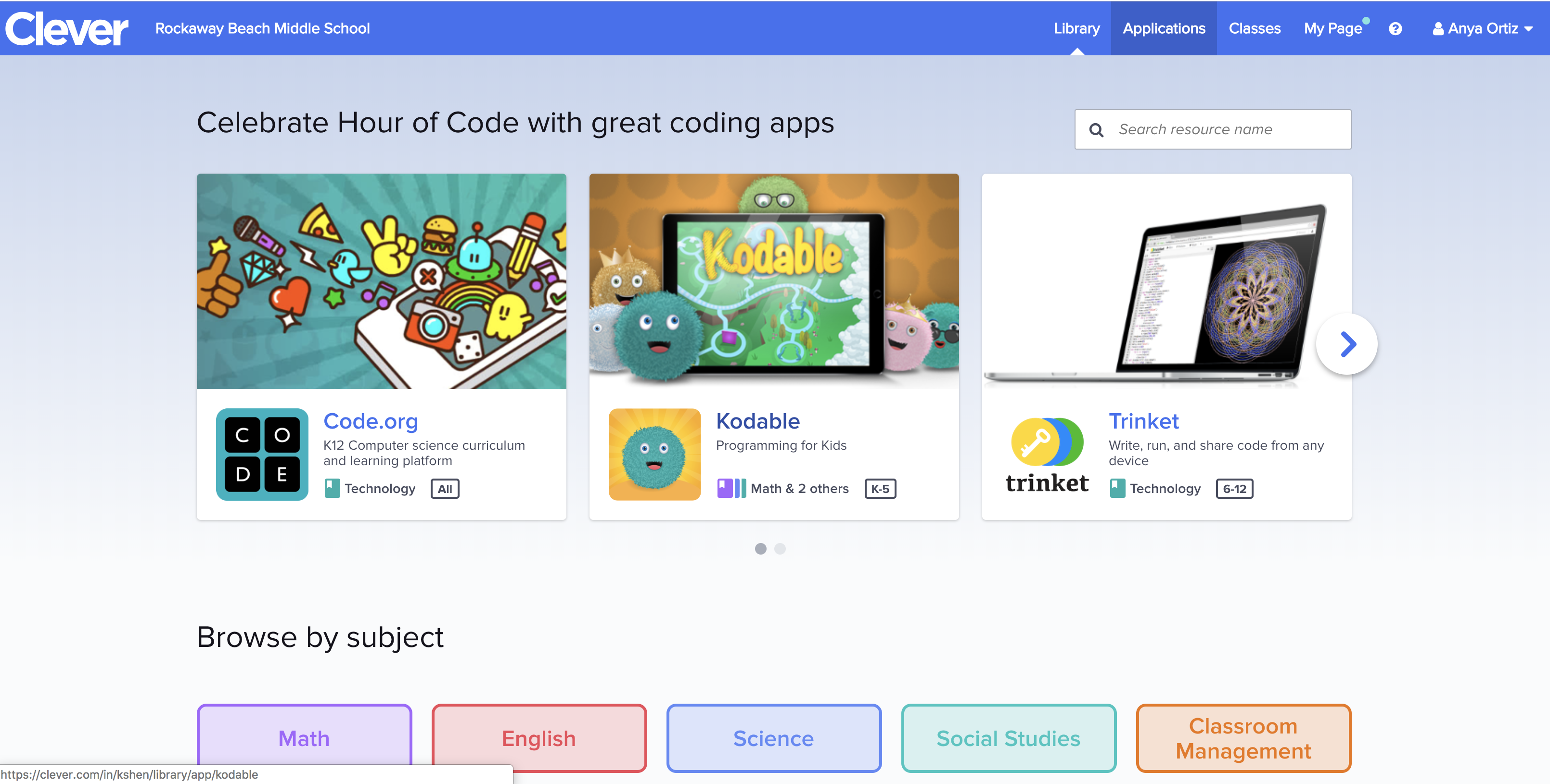This image is from the Clever website, featuring a user interface rich in educational resources. The top navigation bar spans across the width of the screen in a striking blue color, with the word "Clever" prominently displayed in white. On the left side of this bar, there is mention of "Rockaway Beach Middle School," and it includes links to library applications and classes. The user’s profile, identified as Ariana Ortiz, is represented with a question mark icon, and each section has a drop-down menu for additional options.

In the main content area of the website, there is a banner highlighting an event titled "Celebrate Hour of Code with Great Coding Apps." Below this banner, three featured coding apps are displayed for user selection. 

1. **Code.org**: The first app is depicted with a vibrant, multicolored interface, showing various apps emerging from an iPhone. 
2. **Cadoodle**: Appearing to be designed for children, Cadoodle is displayed on an iPad with a child-friendly, playful design.
3. **Trinket**: The final app is shown on a computer and features an image of a flower surrounded by various colors, suggesting its creative and visually engaging nature.

A right arrow indicates more coding apps are available for browsing. Below the featured apps, there are categorized options for users to explore, organized by subject. These include math, English, science, social studies, and classroom management, each represented by distinctively colored icons.